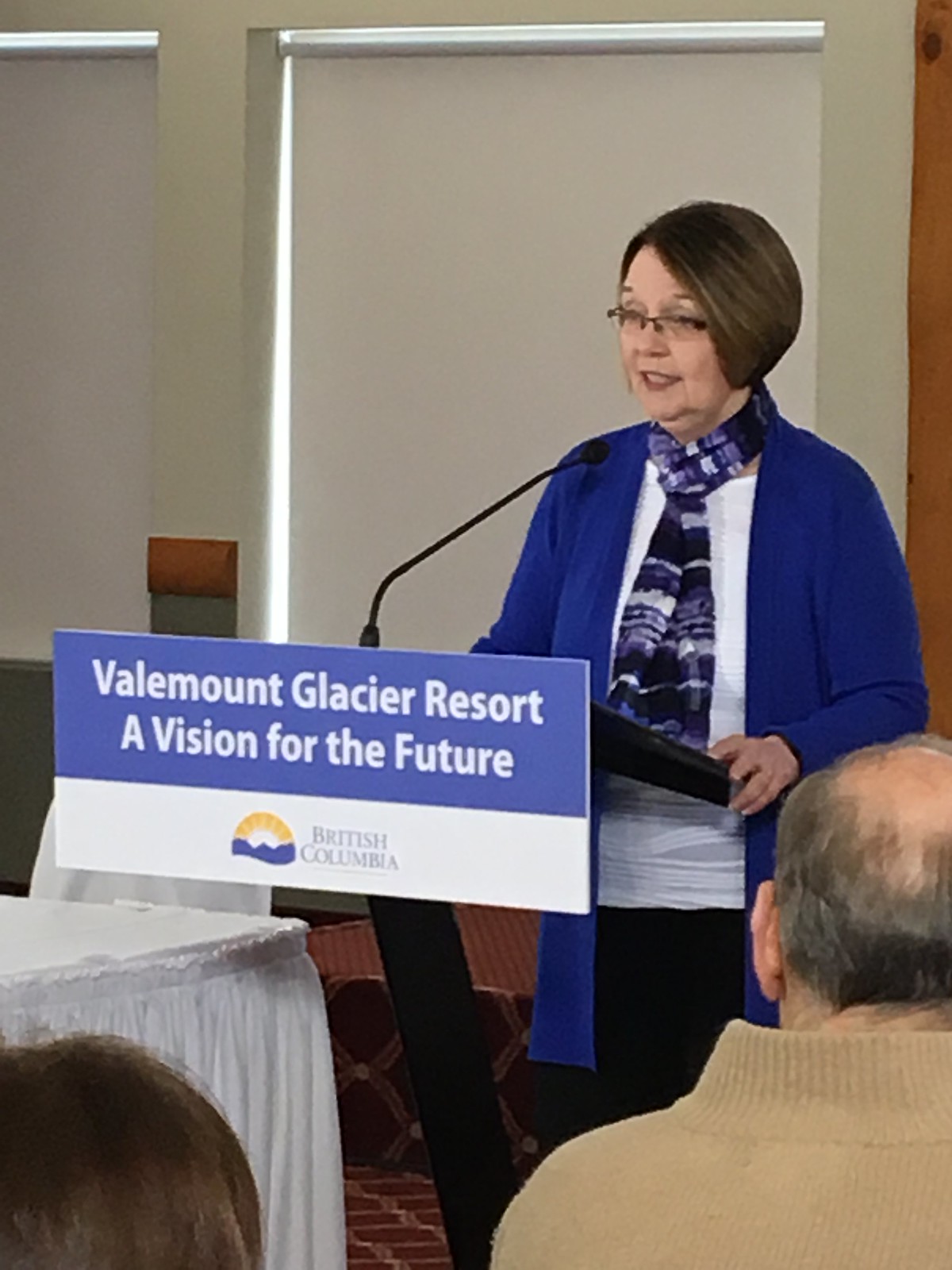The image depicts a woman standing at a black podium equipped with a microphone. She is wearing glasses and has short brown hair. Her attire includes a white t-shirt, a navy blue cardigan, and a dark blue scarf with purple accents draped around her neck. She is facing forward, seemingly addressing an audience. On the podium, there is a poster with a blue background at the top displaying white letters that read, "Valemount Glacier Resort: A Vision for the Future." The bottom portion of the poster is white and features an image of a mountain with a sun over it, adjacent to the text that says "British Columbia" in blue letters. 

In the foreground, we see the back of two audience members, one partially showing a head and a shoulder, while the other reveals only a part of a hand. Behind the woman is a white or beige wall, suggesting they are indoors, possibly in a conference room. Additionally, there is a table on her left, covered with a white tablecloth. There are shades pulled down over the windows, indicating it is daylight outside.